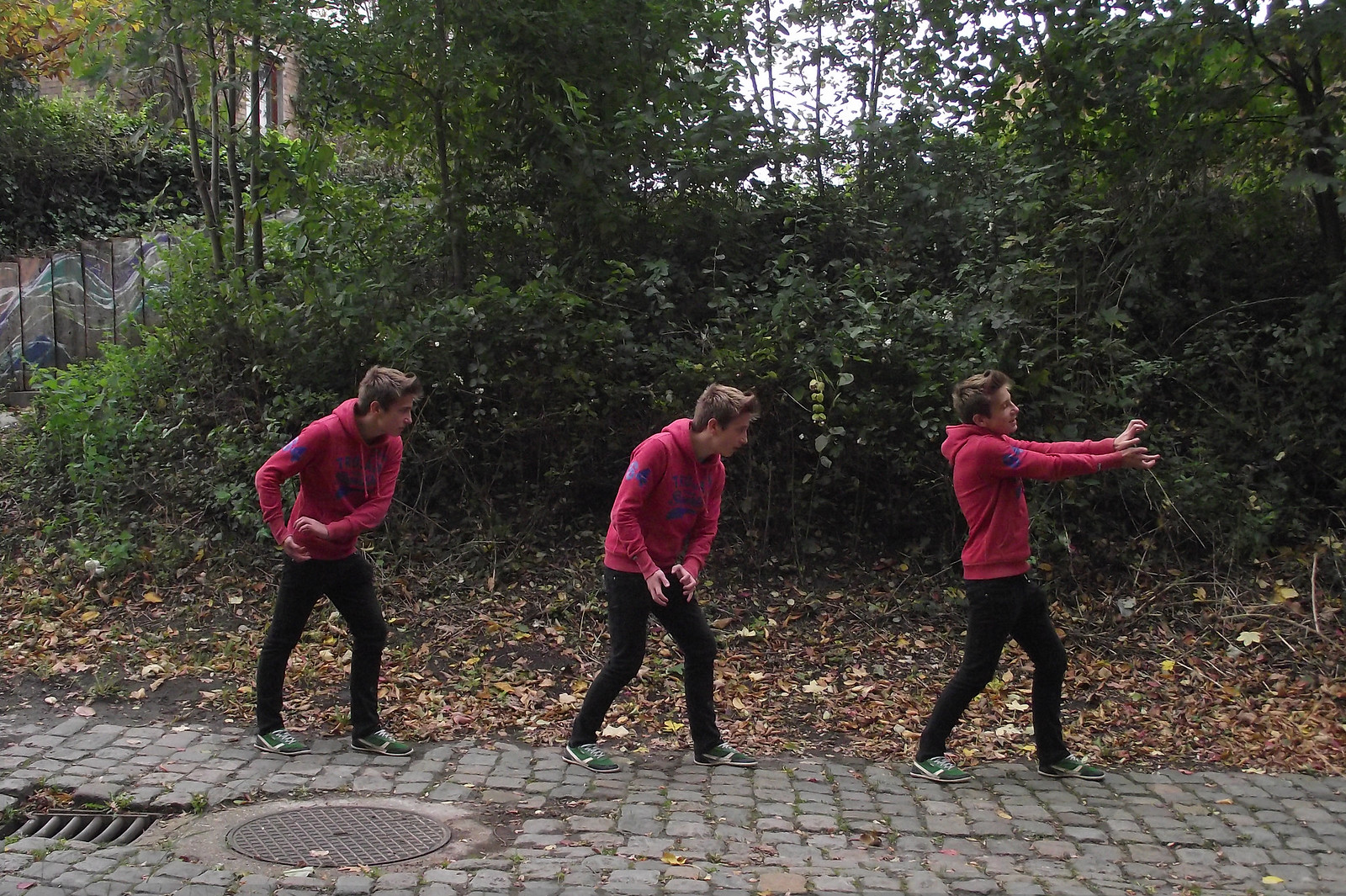In this outdoor, digitally altered color photograph, three images of the same young blonde man are positioned centrally, depicting a sequence of movement. The man, wearing a red hoodie, dark pants, and green sneakers with white stripes, appears to be engaged in an activity involving an imaginary ball. Set against a backdrop of green leafy trees with some brown leaves scattered on the gray cobblestone pathway, the sequence shows the man in different poses: on the left, he holds the imaginary ball near his waist; in the middle, the ball is positioned more centrally; and on the right, he extends his arms forward at chest level as if throwing the ball. A slightly visible white sky peeks through the canopy, and a partially obscured building with a door or window is in the upper left background. Additionally, there's a manhole cover noticeable on the cobblestone pathway.